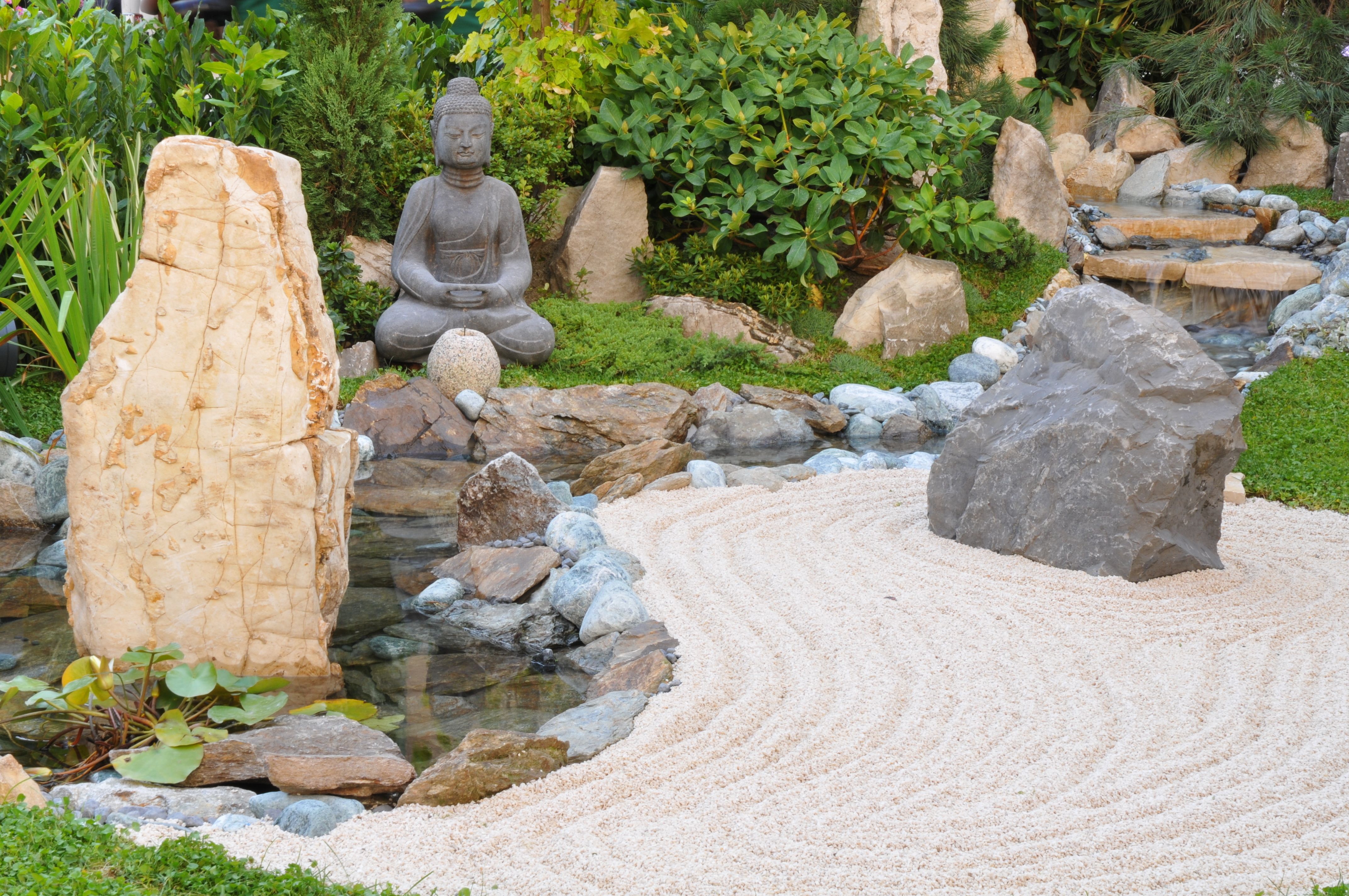The image depicts a meticulously maintained rock garden bathed in daylight. Horizontal and rectangular in shape, the garden is rich with vibrant greenery, featuring an array of shrubs, grasses, and various plants with long and short leaves in shades of dark and light green. Scattered throughout the garden are rocks and stones of different shapes, sizes, and colors, including gray and brown sedimentary rocks.

The centerpiece of the garden is a small, meandering creek that spans from one side of the image to the other, bordered by stones of various hues and forms. Within the creek, there is a prominent, tall, light brown stone resembling a pillar. Flanking the creek on one side is a large gray stone, enclosed by a bed of white sand, reminiscent of a sand garden typically raked into patterns.

In the background, a serene statue of a meditating Buddha, crafted from dark gray stone, sits cross-legged with hands resting in its lap, adding a spiritual element to the tranquil scene. The overall composition of plants, rocks, and water features creates a harmonious and peaceful atmosphere.